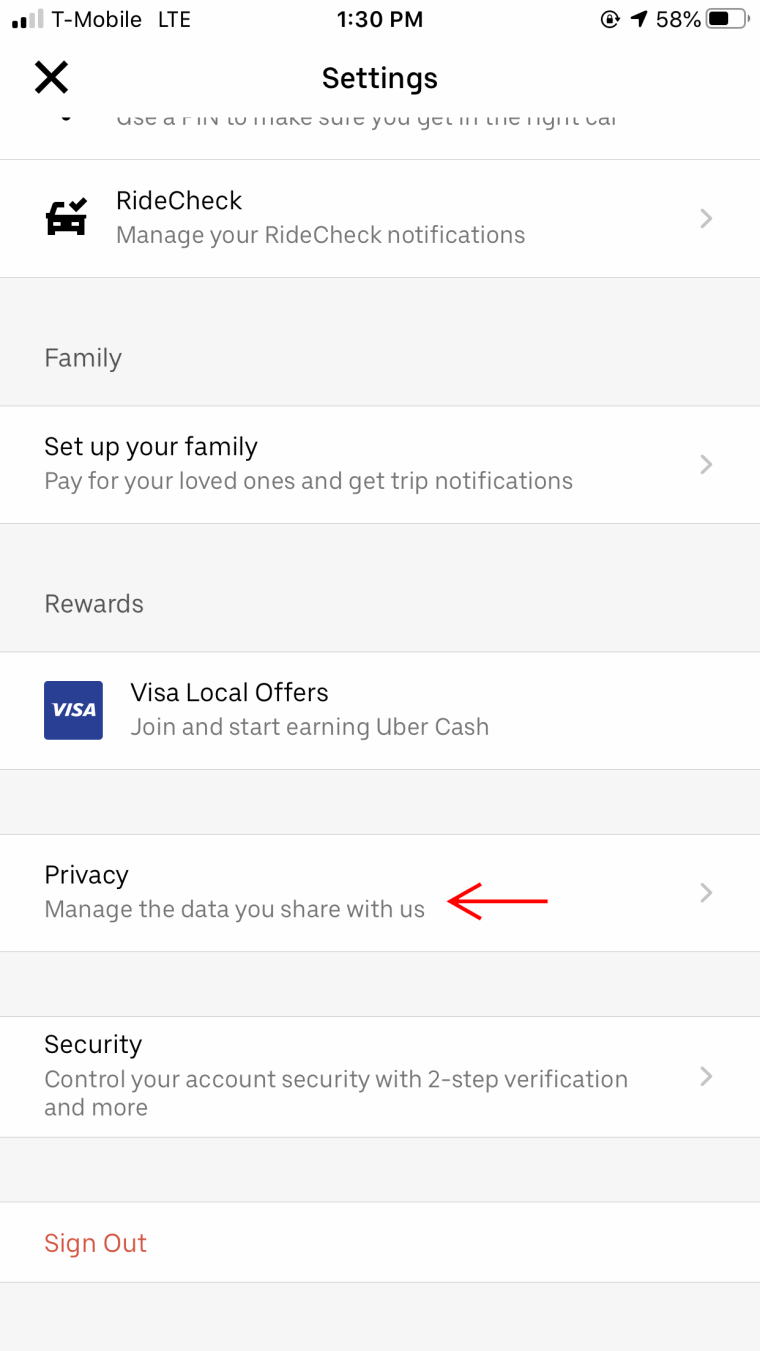Screenshot of a mobile interface displaying settings on a T-Mobile LTE network at 1:30 PM. The status bar shows an airplane mode icon, a circular icon, and a 58% battery charge. Below this, in the top-right corner, there is a black 'X' button to close the settings menu.

The settings page begins with the title "Settings" prominently at the top. Partially visible gray text appears but is cut off, providing little context. 

Here is a detailed rundown of the visible options in the settings menu:

1. **Ride Check**:
   - Icon: Black car with a check mark.
   - Description: "Manage your ride check notifications."
   - Interaction: Contains a gray arrow indicating further options.

2. **Family**:
   - Box Color: Gray.
   - Sub-option: White box with black text.
     - Text: "Set up your family, pay for your loved ones, and get trip notifications."
     - Indicator: Gray arrow pointing right.

3. **Rewards**:
   - Box Color: Gray.

4. **Local Offers**:
   - Box Color: White.
   - Text: "Join and start earning Uber cash."
   - Icon: Navy box with a white Visa logo.

5. **Privacy**:
   - Box Color: White.
   - Text: "Manage the data you share with us."
   - Indicator: Red arrow pointing to the box.

6. **Security**:
   - Box Color: White.
   - Text: "Control your account security with two-step verification and more."

7. **Sign Out**:
   - Box Color: Gray.
   - Text: "Sign out" in red font.

A series of gray and white boxes organize options for easy navigation. The font is large and readable, with a visually appealing, clear, and sharp interface free from any blurring, discoloration, or pixelation.